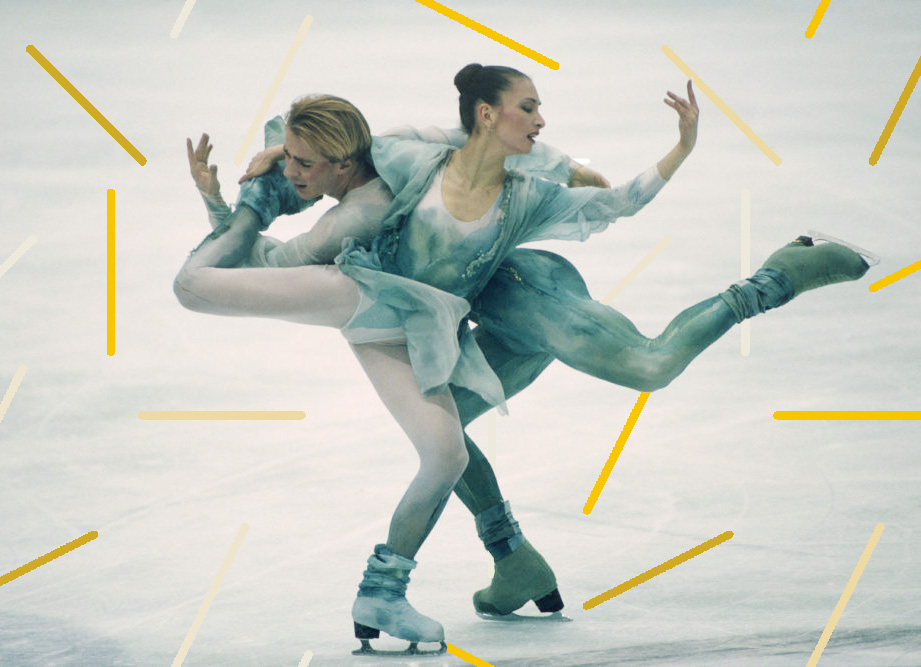The image captures a pair of professional ice skaters, one male and one female, gracefully entwined on the ice, forming a striking central figure. Both skaters are dressed in muted teal blue and white costumes, the male in a snug unitard and the female in a skater skirt outfit. Her hair is elegantly styled in a bun, while his blond hair flows freely. The skaters are executing a complex, balanced spin, with the female’s leg bent and wrapped around the male’s head from the rear. Both are standing on one leg; the male's other leg extends behind him while he raises a hand in a poised ballet pose, mirroring the elegance and strength of the female’s pose. Their synchronized movements and tight embrace emphasize their unity and precision. Decorative yellow stripes float around them, seemingly added post-capture to enhance the dynamic scene. The ice beneath them glistens in stark white, contrasting their teal blue attire and the added yellow elements. Both skaters display visible effort and grace, their blush-highlighted cheeks hinting at the intensity of their performance.